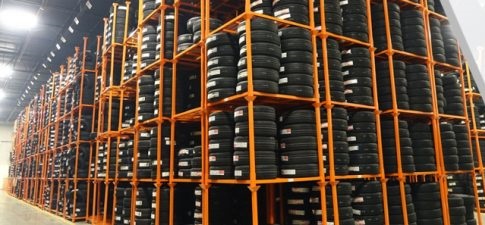The image depicts the interior of a massive tire warehouse featuring an organized grid of orange steel framing units. Each unit consists of square cells capable of holding six black car tires stacked vertically, with each tire clearly labeled. The frames stretch high up, seemingly reaching the ceiling, with rows extending deep into the warehouse on a gray concrete floor. The configuration allows for four sets of six horizontally in each cell, totaling 24 tires per cell. This expansive arrangement, reminiscent of storage seen in large home improvement stores, creates an impression of thousands of tires neatly stored. Overhead lighting illuminates the area, revealing a walkway between the towering stacks of tires. On the left side of the image, the back of the warehouse is visible, while something light gray and dark gray, perhaps an object or part of the structure, is partially clipped on the right side.